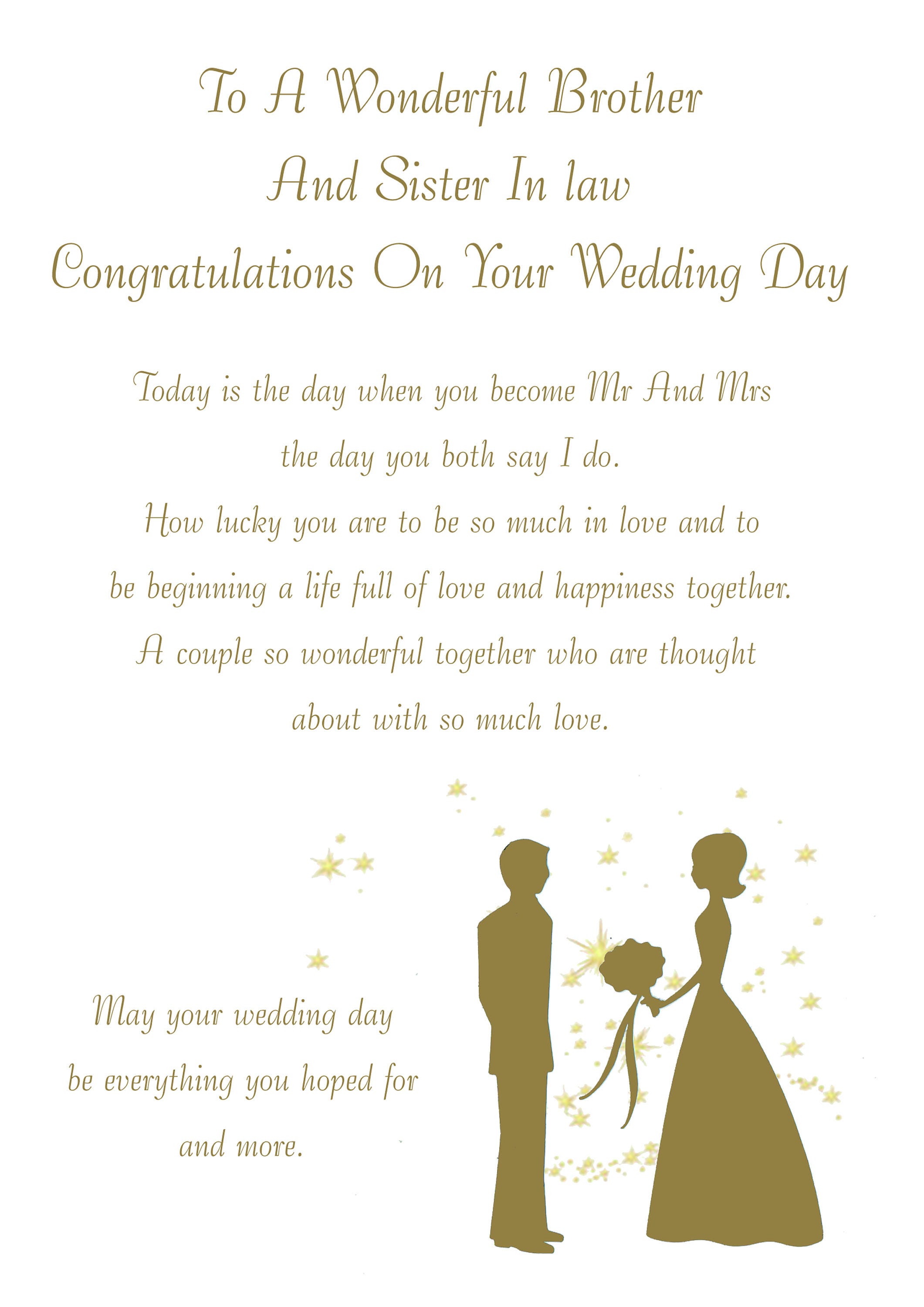This image depicts a wedding congratulations card designed as a vertical rectangle with no visible borders due to its white background matching the background of the card's page. The text is presented in a fancy italic font, some in a larger, gray-colored type. At the top, the card reads: "To a wonderful brother and sister-in-law, congratulations on your wedding day." Below, in centered, smaller font, it continues: "Today is the day when you become Mr. and Mrs., the day you both say 'I do.' How lucky you are to be so much in love and to be beginning a life full of love and happiness together, a couple so wonderful who are thought about with so much love." At the bottom, it concludes with, "May your wedding day be everything you hope for and more." In the lower right-hand corner, there is a dark olive silhouette of a bride and groom, with the bride holding a bouquet.